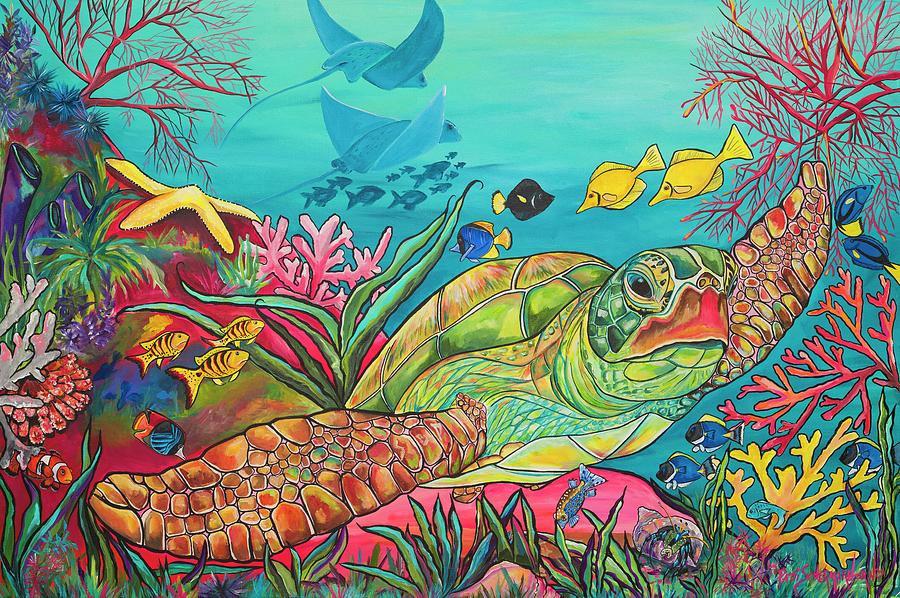This is a highly detailed and vibrant underwater illustration featuring a large sea turtle as its central figure. The turtle, with a greenish-yellow shell, greenish head, and brownish flipper-like arms, is swimming towards the camera, though partially off-frame. The scene is set amidst a colorful coral reef teeming with marine life. The coral varies in vivid shades of pink, blue, green, and red, and is interspersed with green seagrass and numerous fish species in hues of blue, yellow, black, and orange. Nemo-like clownfish in orange and white, as well as blue and yellow fish, add to the lively scene. A starfish is perched on the reef, while a school of bluish fish swims in the background, accompanied by blue stingrays gliding gracefully above. The entire underwater scene is framed by a teal-blue water backdrop, capturing the essence of a bustling, colorful ocean habitat.